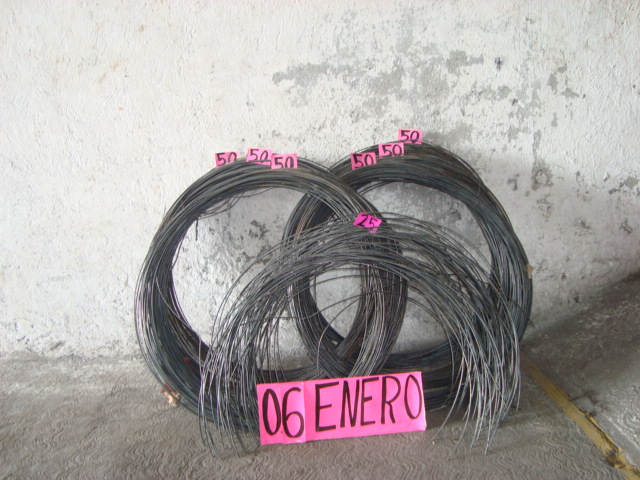This photograph features three coils of metal wire, prominently arranged in the center of the image against a white, slightly scuffed concrete wall. The ground is plain gray concrete that inclines upwards to the right. The coil in the back is slightly offset to the right and has three bright pink sticky notes with "50" written in black text attached. In front of it, and slightly to the left, there is another coil also with three pink "50" sticky notes arranged diagonally. The foreground features a less tightly wound coil in a half-circle shape with a single pink sticky note marked "25". Underneath this coil, a larger pink piece of paper displays "06 enero" in black marker.